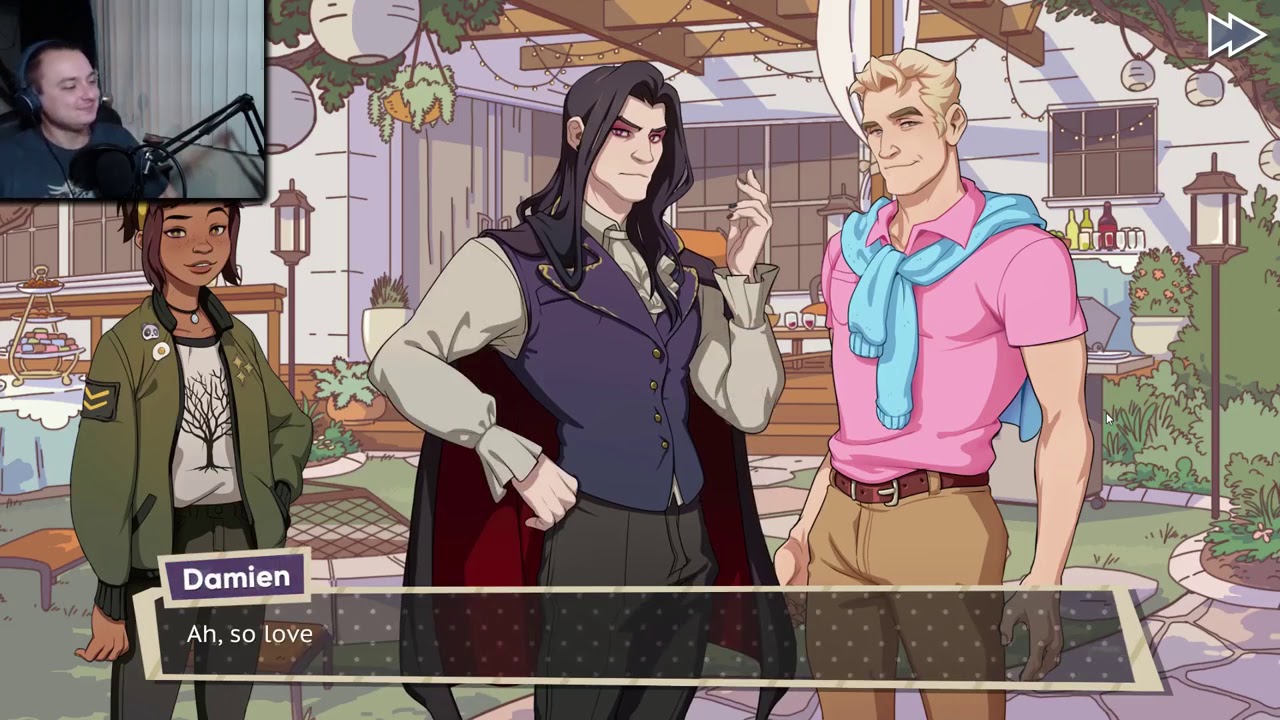In this cartoon or anime-inspired video game image, there are three central animated characters standing on what appears to be a patio, with a well-lit house adorned with party decorations in the background. The first character on the left is a small, female African American wearing a military-style green jacket over a white t-shirt with a tree design. The character in the middle is a tall, pale Caucasian with long black hair, a vampire-like appearance, and is dressed in a purple vest, white puffy shirt, and brown pants. The character on the right is a muscular Caucasian man with blonde hair, wearing a short-sleeved pink shirt, tan khakis, and a turquoise scarf draped over his neck. In the top-left corner of the image, there is a photorealistic inset of a Caucasian man with headphones and a microphone, positioned in front of white curtains, suggesting he's streaming or commenting on the game. At the bottom of the main image, a text box displays the name "Damien" in a smaller box and the line "Ah, so love" in a larger box, indicating this is part of a dialogue from the game.